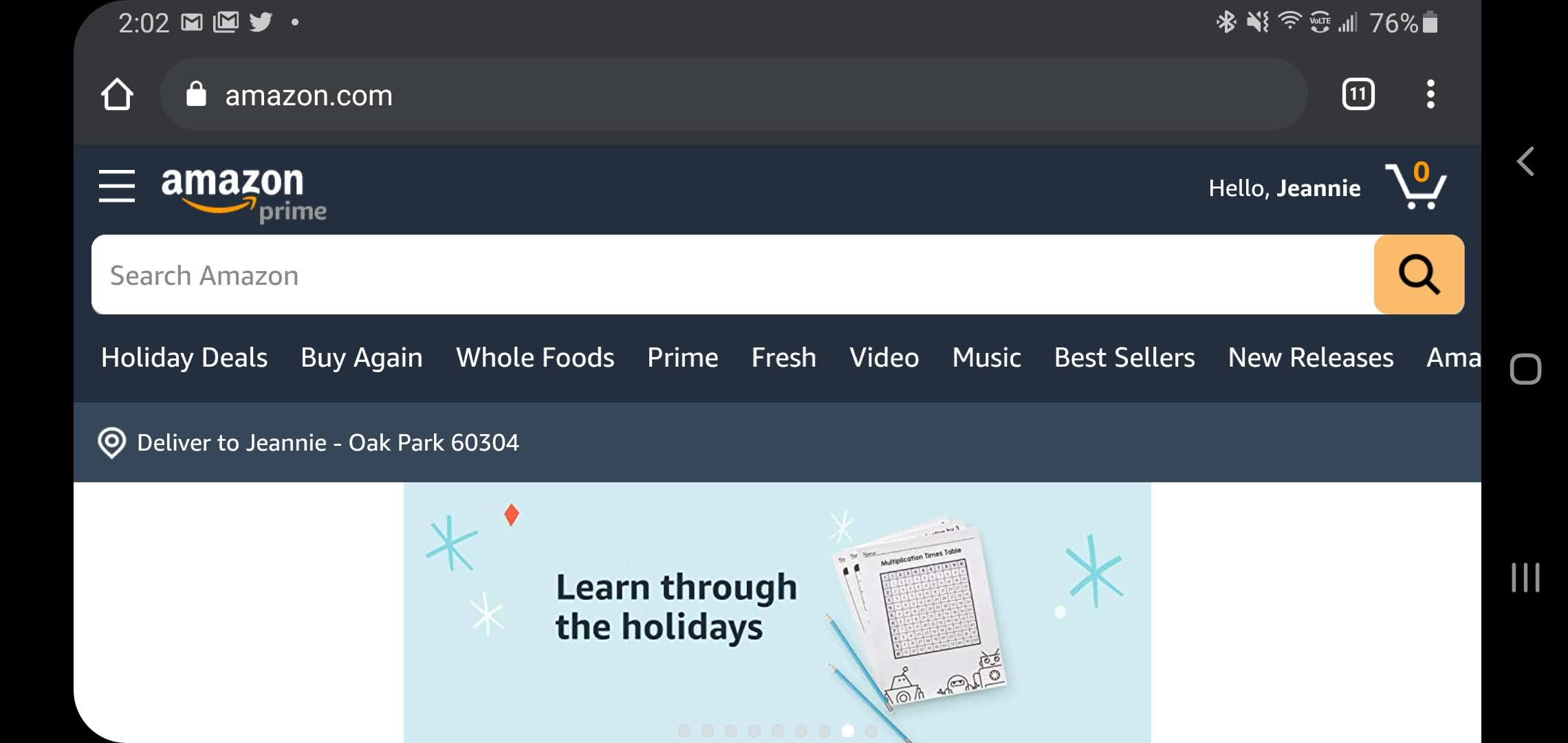A screenshot of the Amazon website is displayed at 2:02 PM, showing various interface elements. In the browser's address bar, "https://www.amazon.com" is marked with a padlock icon, indicating a secure connection. The interface includes multiple icons to the right, such as Gmail and Twitter, followed by indicators for strong Wi-Fi, Bluetooth connectivity, and a phone battery at 76%. At the top of the webpage, the Amazon Prime logo is displayed next to a greeting, "Hello, Janine," with her shopping cart showing zero items. Below, there is a distinct gray rectangular textbox displaying "amazon.com" in lowercase. Directly underneath is a search bar in white, featuring a magnifying glass icon for search, followed by various shopping categories like Holiday Deals, Buy Again, Whole Foods, Prime Fresh, Video, Music, Bestsellers, and New Releases. The delivery address is specified as "Delivered to Janine Oak Park 60304."